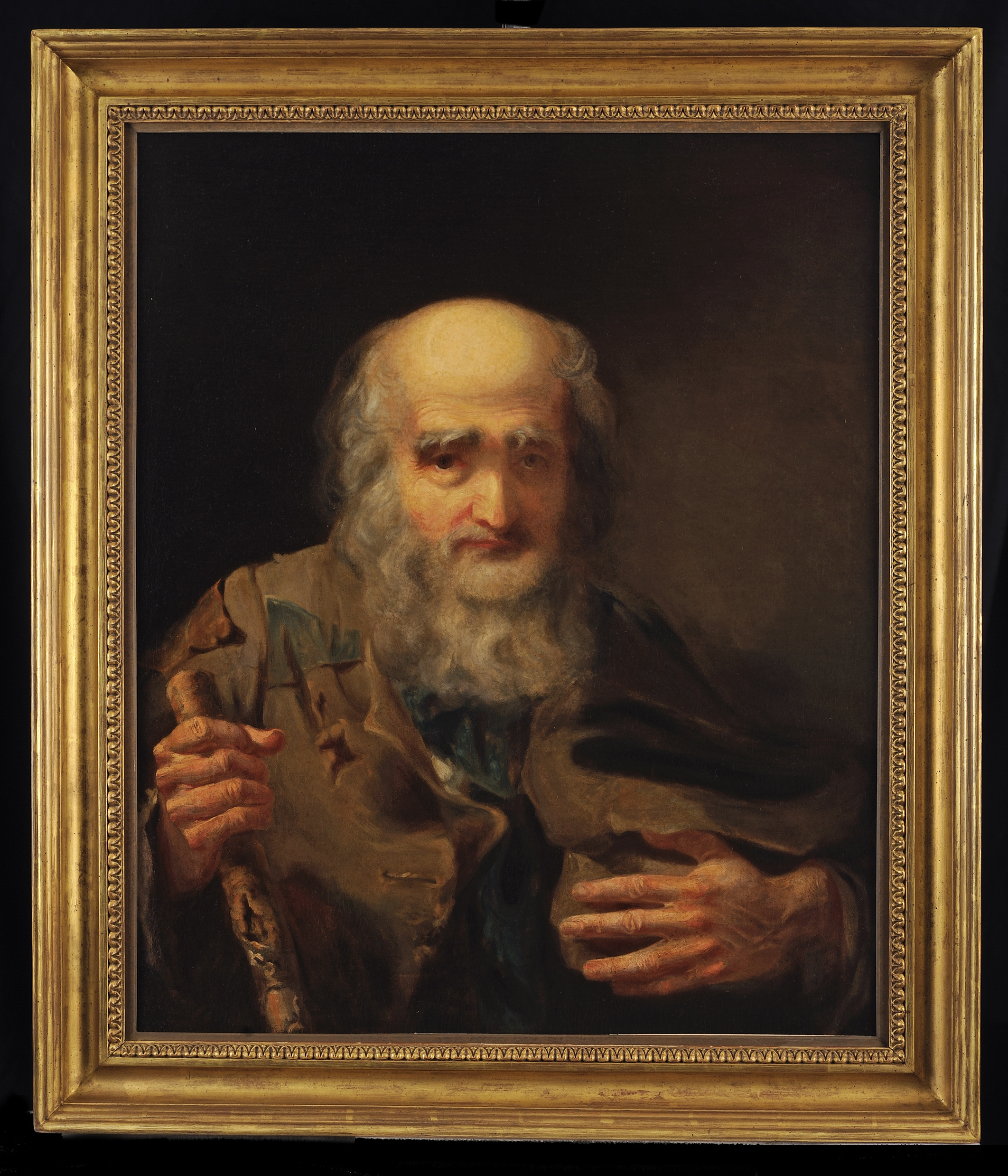This painting, enclosed in a rectangular frame measuring approximately six inches high by five inches wide, features a detailed portrayal of an elderly gentleman. The frame has a thin black border, with the wood painted in ornate bronze-brown or gold, highlighting intricate design details near the picture. The man in the painting appears to be in his 70s and is depicted from mid-chest up as he looks directly at the viewer with dark brown eyes. His expression is neutral, possibly with a slight grin, giving the impression of a thoughtful, yet serene demeanor.

He is bald on top, with white and gray curly hair cascading down the sides of his head, blending seamlessly into a long, thick beard that extends down to his chest. His eyebrows are bushy and thick, almost overshadowing his eyes, and the deep wrinkles on his forehead add to his aged appearance. The man's attire is a worn, green jacket adorned with patches—brown on his right shoulder and a darker green on his chest—and he wraps himself with a grayish-colored scarf. 

In his left hand, partially concealed by his jacket, he holds what appears to be a hat, while his right hand grips an old wooden cane or walking stick. The background of the painting transitions from a dark black to a grayish-brown hue, framing the figure with a subtle contrast that enhances the depth of his character. Overall, the painting exudes an aura of quiet wisdom and resilience, beautifully captured by the artist's meticulous attention to detail.